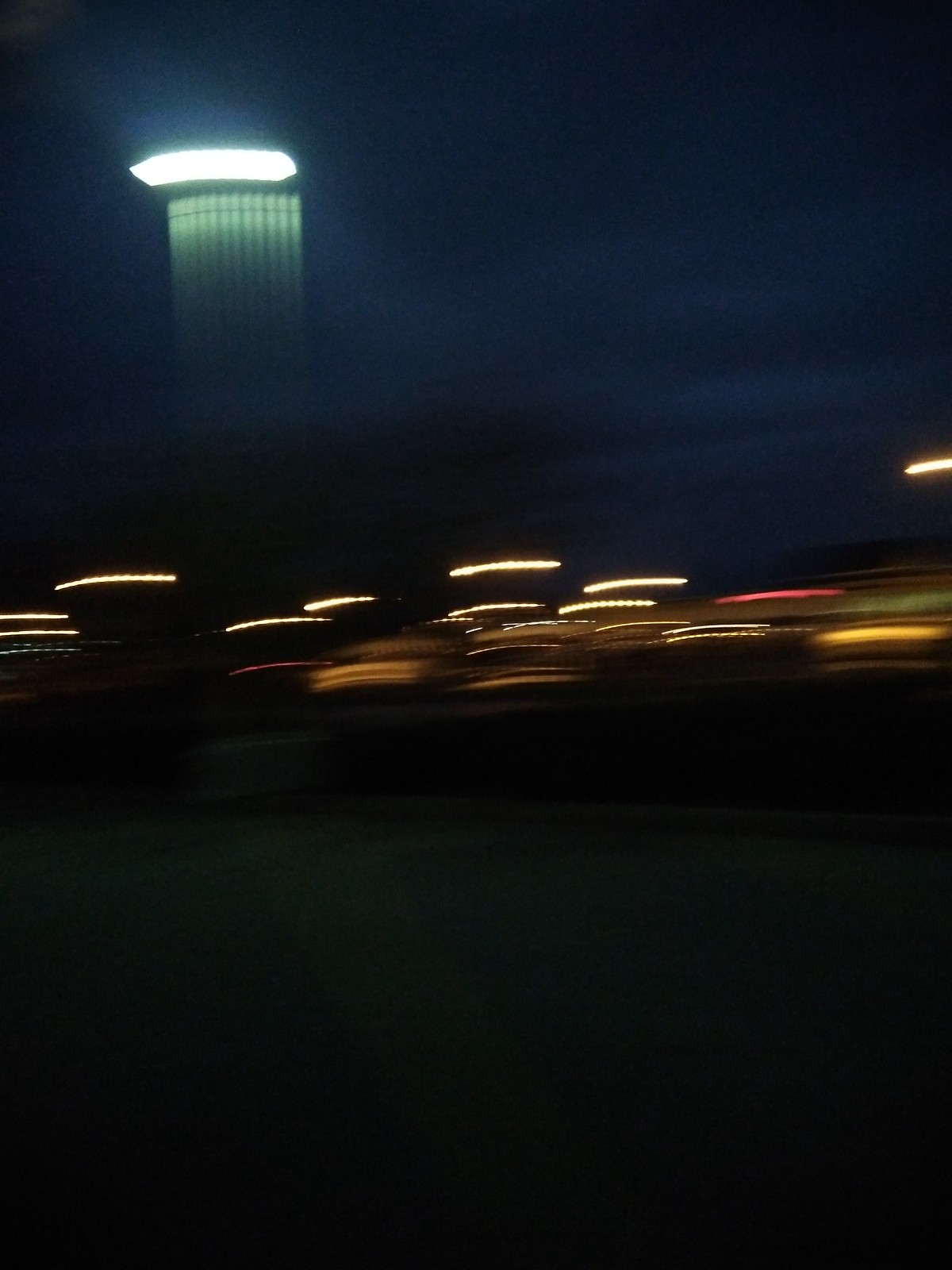The image captures the blurred interior view from a car window at night, with the road ahead rendered incredibly hazy due to the vehicle's high speed. Dominating the center of the image are elongated, stretched lights in whites, yellows, and reds, forming horizontal and slightly curved lines against a predominantly black lower half. Near the top left corner, the dark expanse reveals a faintly visible streetlight or possibly a floodlight with an oval beam, producing multiple ghostly vertical poles due to motion blur. Above the chaotic interplay of lights, the sky transitions from a very dark blue to black, dotted with cloud-like shapes, adding depth to the nighttime scene. The overall effect is one of rapid movement and distortion, vividly capturing the sensation of speed and darkness.